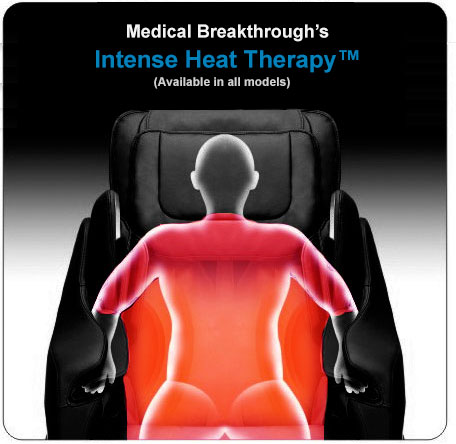The image is a square with rounded corners, featuring a central black cushioned chair with armrests against a gradient background that transitions from solid black at the top to gray in the middle and white at the bottom. At the top of the image, white text reads "Medical Breakthroughs," followed by "Intense Heat Therapy" in blue, and a parenthetical note in white, "Available in all models." A digital representation of a person is displayed leaning forward into the chair, their hands in visible compartments. The person’s outline glows with red and orange hues, suggesting intense heat therapy focusing on their torso, while a grayscale outline highlights their head. This advertisement, which features a trademarked term for "Intense Heat Therapy," evokes a professional, medical aesthetic, suitable for a doctor's office poster.